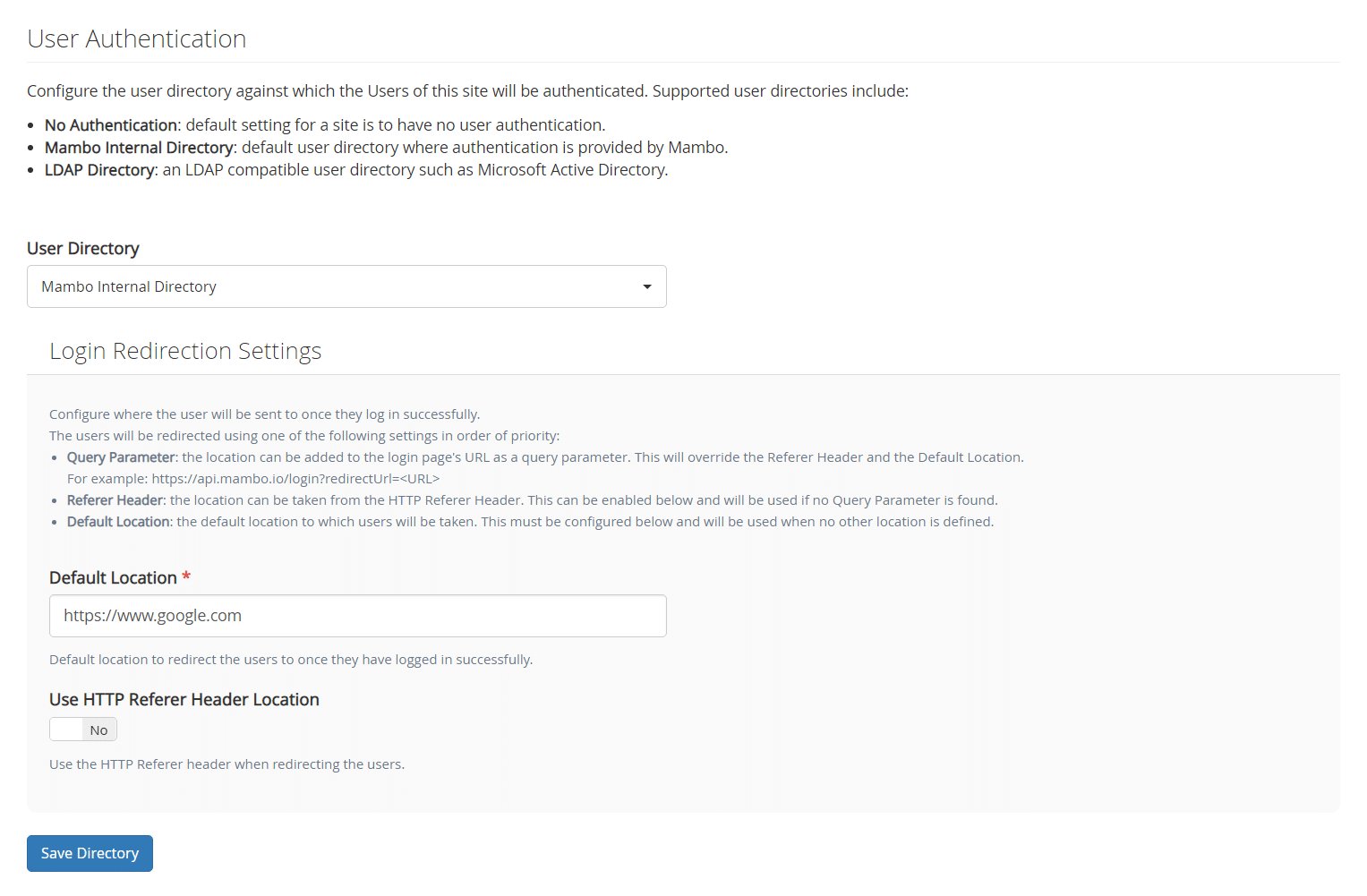This image displays a user authentication screen. At the top left, the title "User Authentication" is clearly visible. Below this title, there's a description instructing the user to configure the user directory for site authentication. It details that supported user directories include "No Authentication," "Mambo Internal Directory," and "LDAP Directory." 

Currently, the "User Directory" is set to "Mambo Internal Directory." Further down, the "Login Redirection Settings" section contains six lines of very small text. Within this section, six crucial terms are highlighted: "Query Parameter," "Refer Header," and "Default Location." Under the "Default Location" heading, there's a URL input field containing "www.google.com," with the input bar appearing white.

Additionally, there is an option labeled "Use HTTP Refer Header Location," followed by a white checkbox and a "No" option in a gray box. Beneath these options, a very small line is seen.

At the bottom left corner of the image, there's a blue button labeled "Save Directory." The screen is divided into two color schemes: the bottom half has a light gray background, while the top half features a white background surrounding the text.